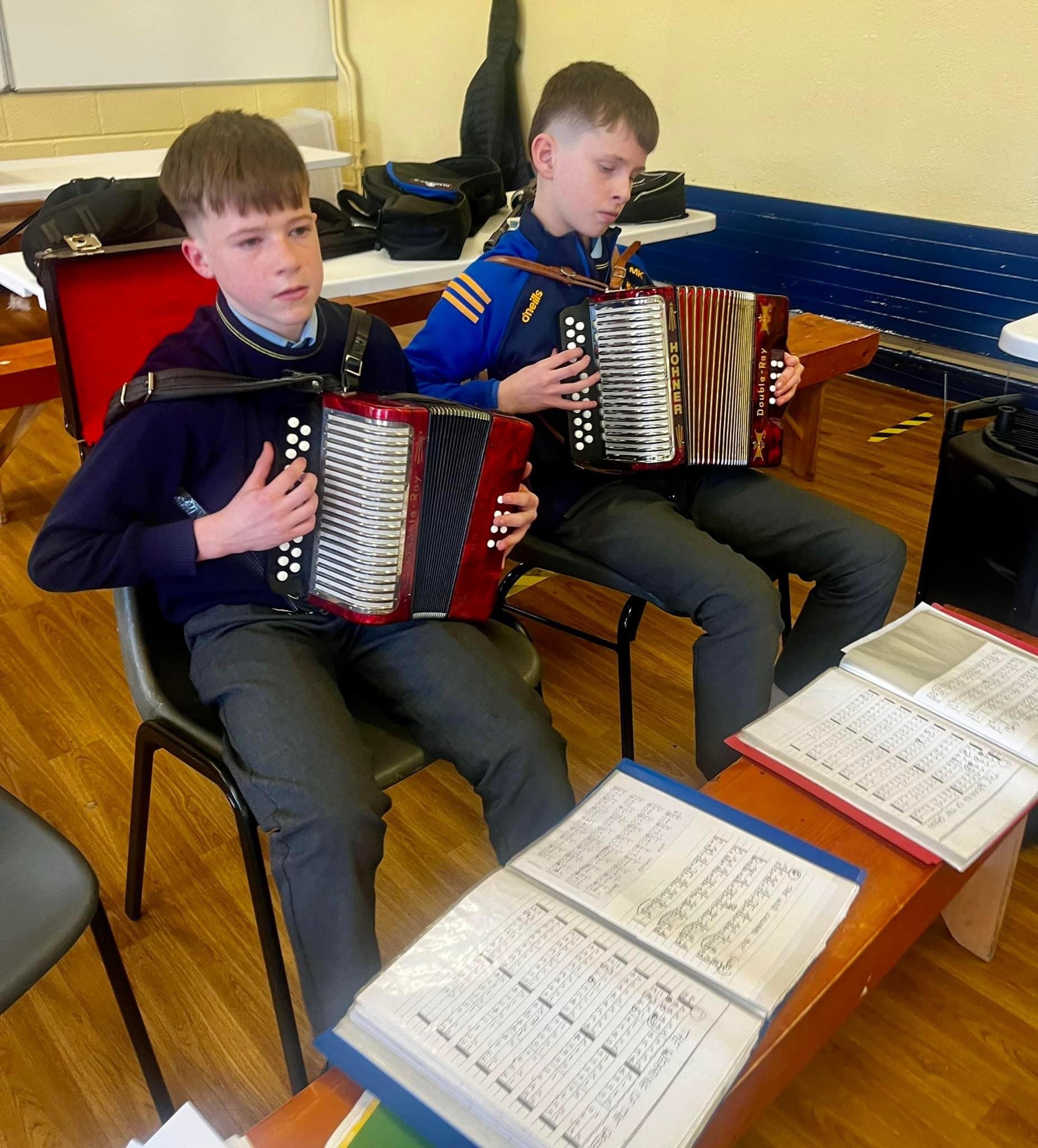In this photograph, two boys, approximately 12 years old, are seated in chairs within a room featuring a hardwood floor and yellow walls. In front of them is a wooden table displaying accordion music sheets spread out in a notebook format. Both boys are playing red accordions and are intently looking forward, slightly downward. They each have short brown hair and are dressed in long sleeves and dark grey pants. One boy wears a blue sweater over a collared shirt, while the other sports a blue Adidas jacket labeled "O'Neal’s". Also visible in the room is a black backpack, suggesting a school setting, possibly a music room.